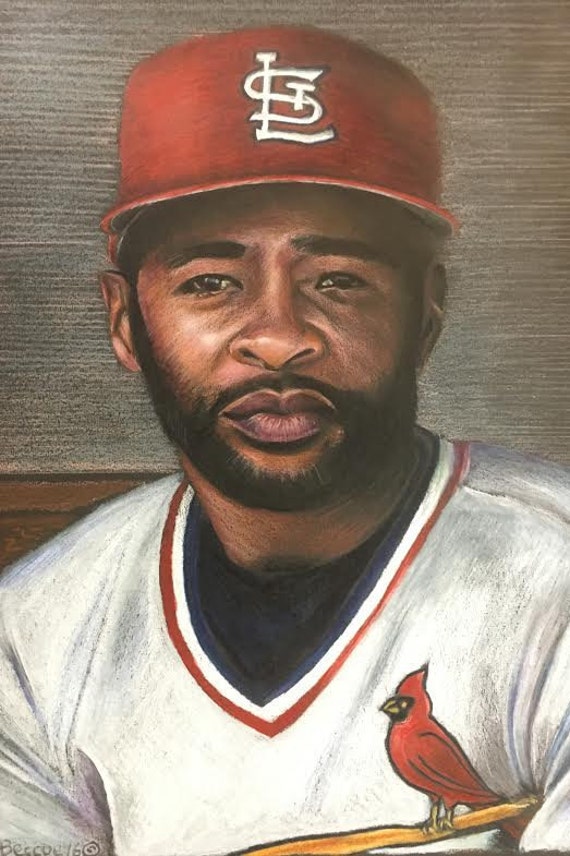This detailed, highly realistic illustration depicts an African-American man, possibly a St. Louis Cardinals baseball player, who sits posed and gazes directly at the viewer with slightly squinted eyes. He dons a red St. Louis Cardinals baseball cap featuring the white interlocked "SL" logo and a full beard. His attire includes a white Cardinals jersey adorned with a red Cardinal perched on a bat across the chest, beneath which he wears a black shirt. The image, skillfully rendered with either charcoal, colored pencil, or pastel, captures the player's composed demeanor as if drawn from a photograph.